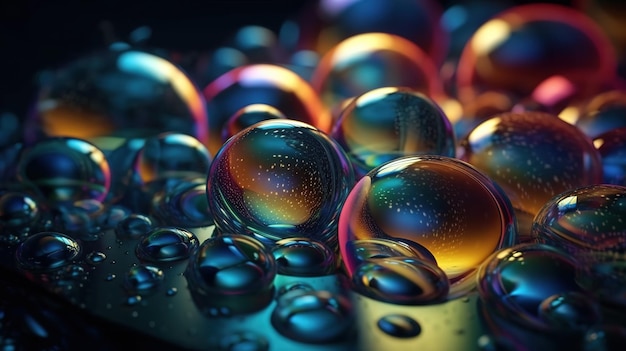This photograph captures a stunning arrangement of vibrant, luminous bubbles against a black, almost leather-like surface. The image, seemingly taken in the dark with a spotlight, creates a beautiful contrast that emphasizes the ethereal quality of the bubbles. The bubbles vary in size, from grape-sized to raindrop-sized, filling the entirety of the rectangular frame. These transparent, prism-like bubbles display a spectrum of colors—pink, blue, orange, yellow, green, and dark purple. The bubbles in the foreground are in sharp focus, exhibiting a metallic blue sheen that makes them look like gems, while those in the background blur out, creating a depth effect. The light reflections on the bubbles range from bright and vivid on the larger bubbles to more subtle on the smaller ones, creating a mesmerizing display of iridescence. This beautiful composition captures the delicate and transient nature of bubbles, making them appear both tangible and otherworldly.